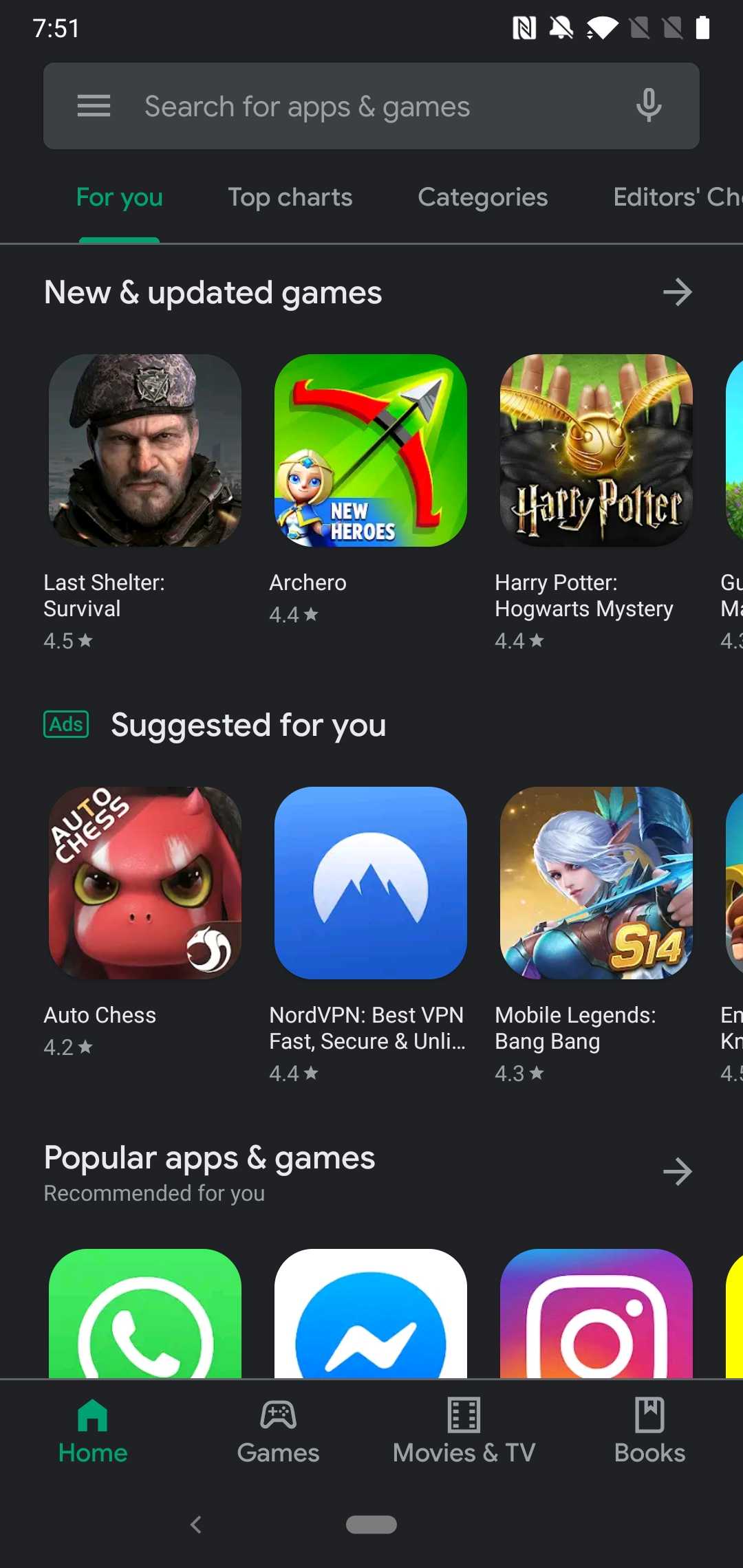This image is a screenshot of a mobile app store interface. The background at the top is predominantly black with white text, highlighting the current tab in green text. The menu bar at the top lists various sections: "For You," "Top Charts," "Categories," "Editor's Choice," with the last part of the menu faintly visible and cut off. Below the menu bar is the "New and Updated Games" section, featuring a selection of games such as "Last Shelter," "Archero," and "Harry Potter." Underneath this section, there's a "Suggested for You" category displaying apps like "Auto Chess," "NordVPN," and "Mobile Legends." Further down, there's a "Popular Apps and Games" section where recognizable apps such as "Google Voice," "Messenger," and "Instagram" are visible. At the bottom of the screen is a footer with several icons indicating different sections of the app store: "Home" (which is currently selected and highlighted in green), "Games," "Movies & TV," and "Books," all in white text.